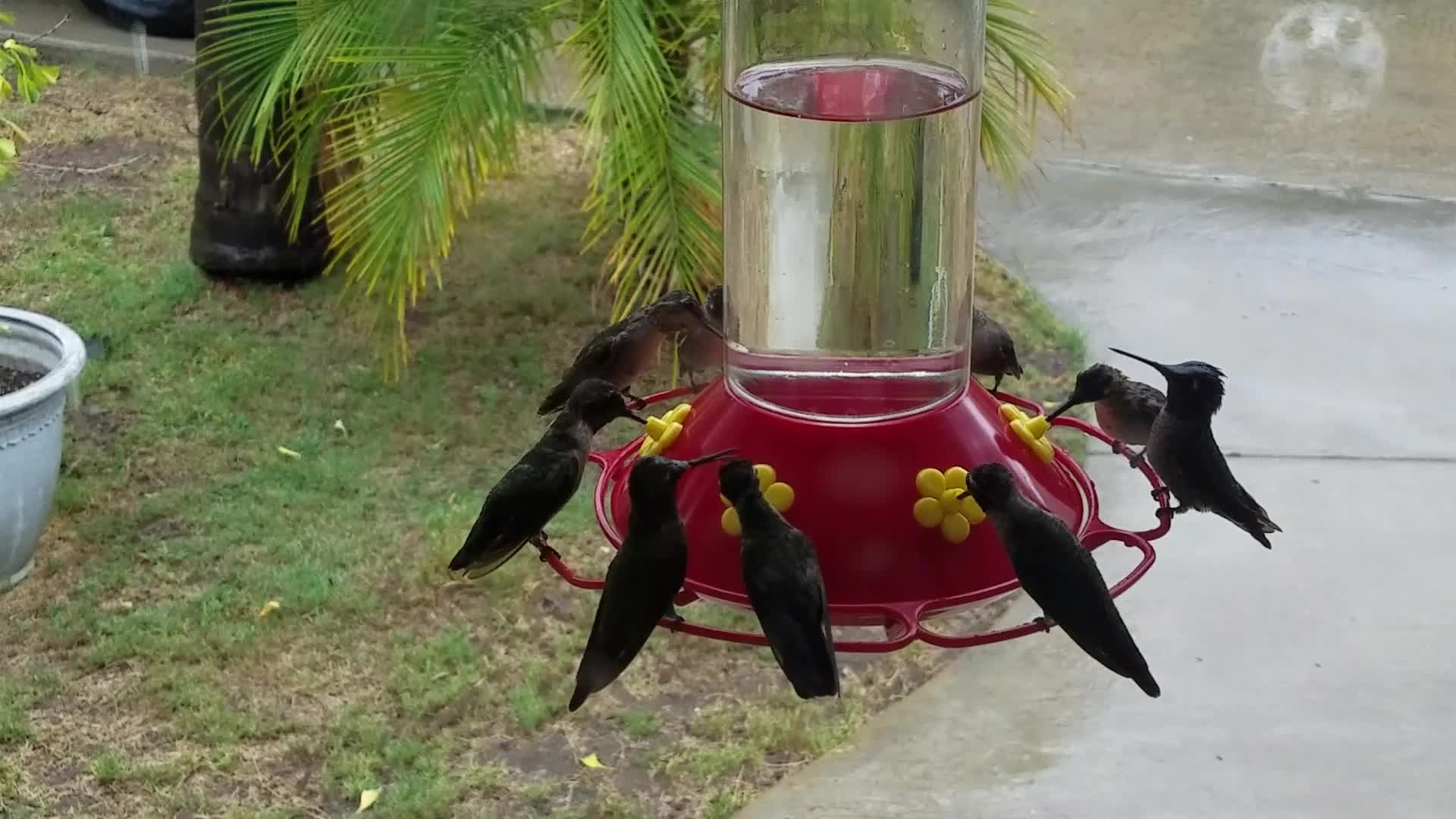The image depicts a busy hummingbird feeder, prominently featuring a clear, cylindrical container filled halfway with clear liquid, likely nectar. The feeder has a red, flared-out plastic base adorned with six yellow plastic flower shapes arranged around its perimeter, from which the birds drink. Surrounding the base are thin red plastic perches. The feeder is entirely encircled by nine hummingbirds, all black with a slight greenish tint, either feeding from the flowers or perched, waiting their turn. The background showcases a lush yard with vibrant green grass, a palm tree, and a curved, wet cement pathway. A cement planter is visible on the left side of the photograph.